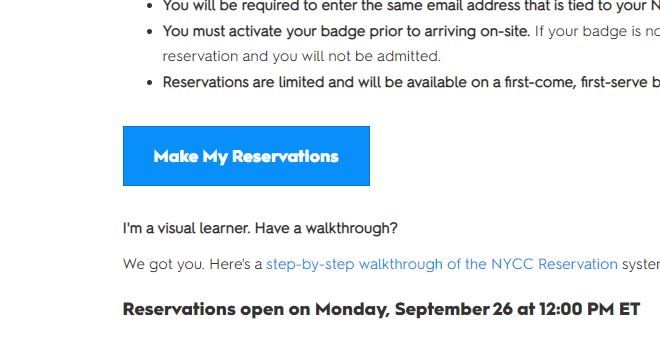The image displays detailed instructions on a computer screen, specifically related to making reservations, presumably for an NYCC event. At the top of the screen, there are three bullet points with important information:

1. The first bullet point begins with "You will be required to enter the same email address that is tied to your..." but the rest of the text is cut off.
2. The second bullet point starts with "You must activate your badge prior to arriving on site if your badge..." and it's partially cut off. It appears to continue on the next line with "reservation, and you will not be admitted."
3. The third bullet point states "Reservations are limited and will be available on a first-come, first-serve..." but again, the complete sentence is cut off.

Below these bullet points, there is a large blue rectangle featuring the text "Make My Reservations." Beneath this button, there is a message that reads, "I'm a visual learner. Have a walkthrough? We got you. Here's a step-by-step walkthrough of the NYCC reservation system." The phrase "step-by-step walkthrough of the NYCC reservation" is blue and appears to be a clickable link, likely directing users to additional instructions or a video guide.

At the bottom of the image, there is a note in dark black text saying, "Reservations open on Monday, September 26 at 12 PM ET." The overall background of the image is white, providing a clean and clear layout for the text and elements displayed.